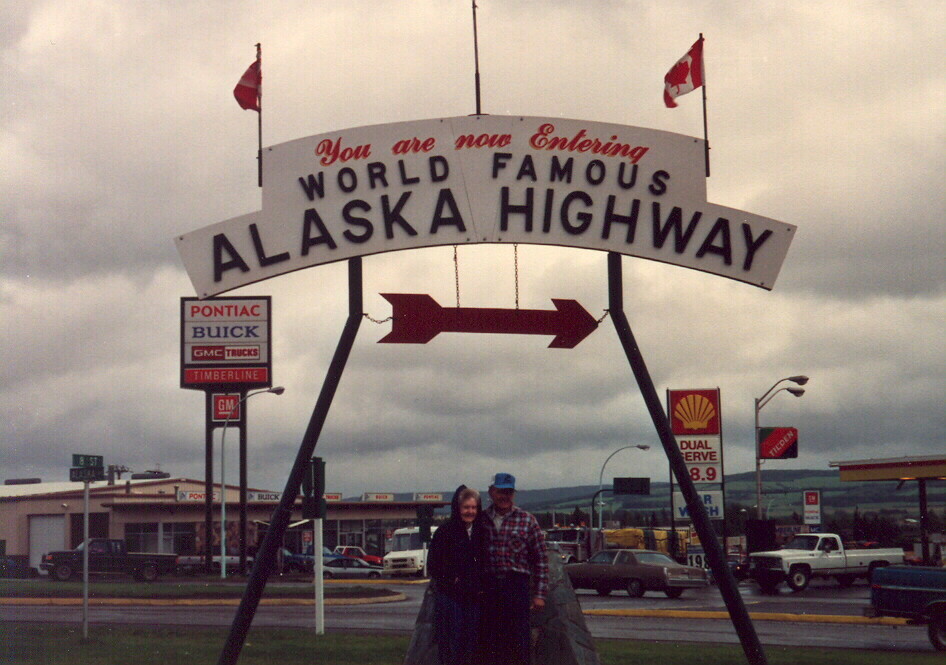In this full-color daytime photograph, a cloudy, overcast sky looms overhead, suggesting recent rain. The central focus is a large, white sign with red and black lettering that reads, "You are now entering world-famous Alaska Highway," accompanied by a red arrow pointing to the right. Below the sign sits an elderly couple, the woman in a dark blue hooded sweatshirt and blue jeans, the man in a plaid shirt and blue trucker hat. They appear to be sitting in front of a large rock, with the woman holding the man. 

In the background, there is a Shell gas station to the right and a Pontiac, Buick, GMC Trucks dealership to the left, indicating "Timberline GM." Several vehicles, including a couple of white trucks, a blue car, and a brown car, are scattered around. The scene is busy with multiple roads, medians, and more parked vehicles visible. The overall atmosphere is nostalgic and serene, capturing a slice of everyday life at the entrance to this historic highway.